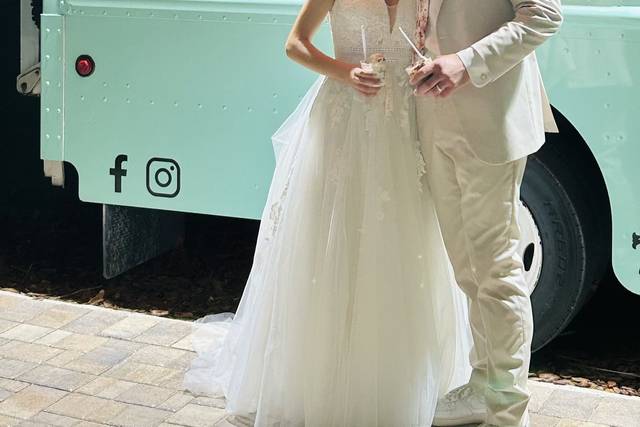This image captures an outdoor scene featuring a bridal couple from mid-chest down to their legs. The groom is dressed in an all-white ensemble, including a white suit jacket, shirt, pants, and sneakers. The bride wears a white, sleeveless wedding dress with a long tulle skirt reaching the ground. They stand close to each other, holding clear plastic cups with white spoons, likely filled with ice cream. The bride’s other arm is wrapped around the groom. Their backdrop includes a faded pastel blue or teal vehicle, which appears to be an ice cream truck with symbols indicating Facebook and Instagram. The truck is partially visible, showing a side light, and black tires, and is parked on a street next to a brick sidewalk where the couple stands. The setting appears to be taken outside, though it is unclear whether it is daytime or nighttime. The color palette of the image includes off-white, white, black, mint green, teal, red, tan, and light gray.